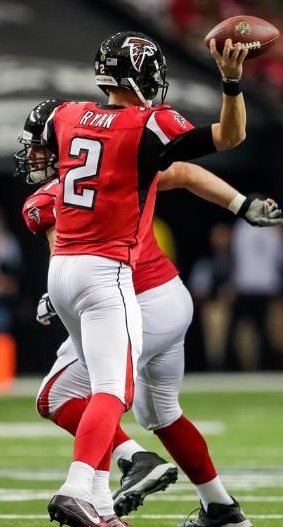In the photograph, two football players from the Atlanta Falcons are captured during a game on the field. Both athletes are dressed in matching uniforms—red and black on the tops, white pants, red socks, and black helmets adorned with an eagle emblem. The player in the foreground, identified by the name "Ryan" and the number 2 on his back, is about to throw a brown football with his right hand. His stance is poised, with his back facing the camera. In the background, another player appears to be running or turning, bent slightly at the knees, with one arm visible beneath Ryan's throwing arm. The green field with white markings is noticeable beneath their feet, while the upper background is a blur of colors—orange, yellow, white, black, and red—indicating the presence of spectators and the dynamic atmosphere of the game.